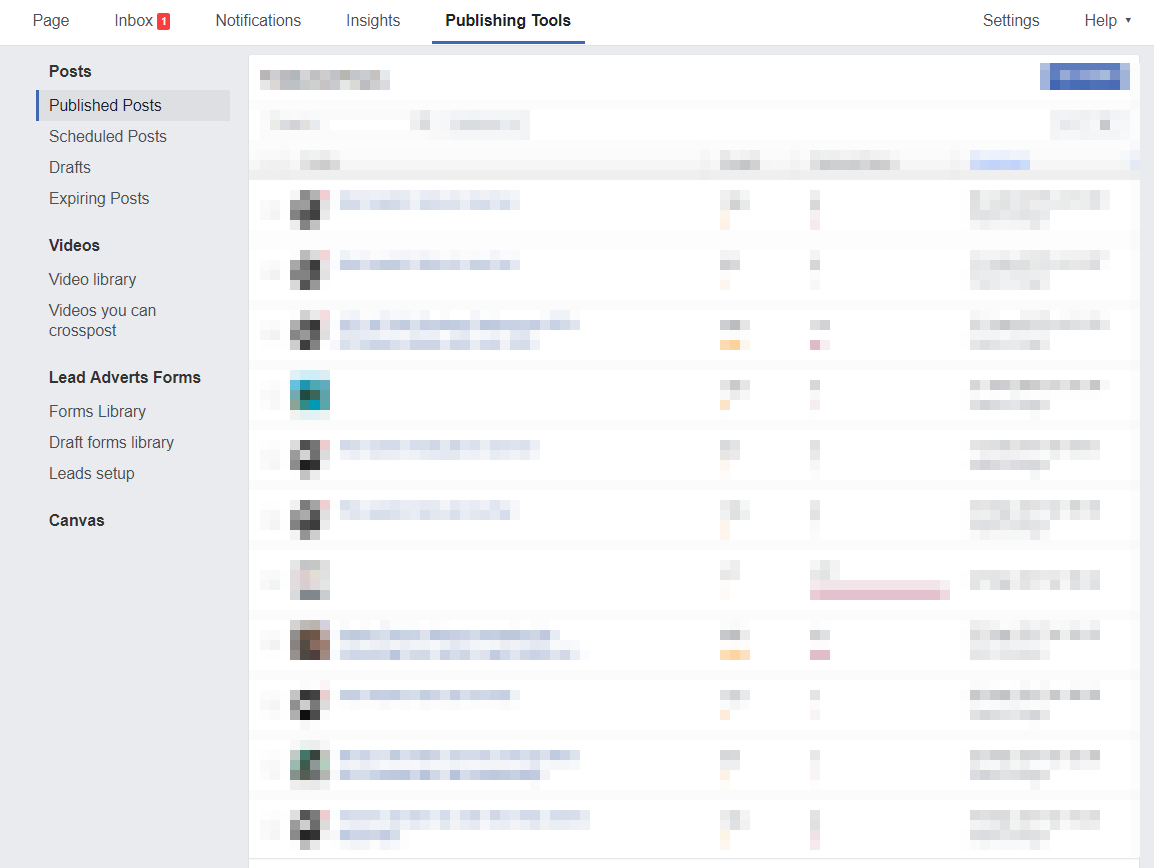The image is a screenshot of a website interface where the majority of the content is blurred, leaving only the headings and navigation tabs visible. At the top, a set of main sections or tabs are displayed, starting from the left with "Page" followed by "Inbox," which has a red notification box containing the number one. The subsequent tabs are "Notifications," "Insights," and "Publishing Tools." On the left-hand side, there is a sidebar with alternate tabs for various post and media management options, including "Post," "Published Posts," "Scheduled Posts," "Drafts," "Expiring Posts," "Videos," "Video Library," "Videos You Can Crosspost," "Lead Adverts Forms," and "Form Library." The screenshot captures the structural layout and navigational elements of the website.